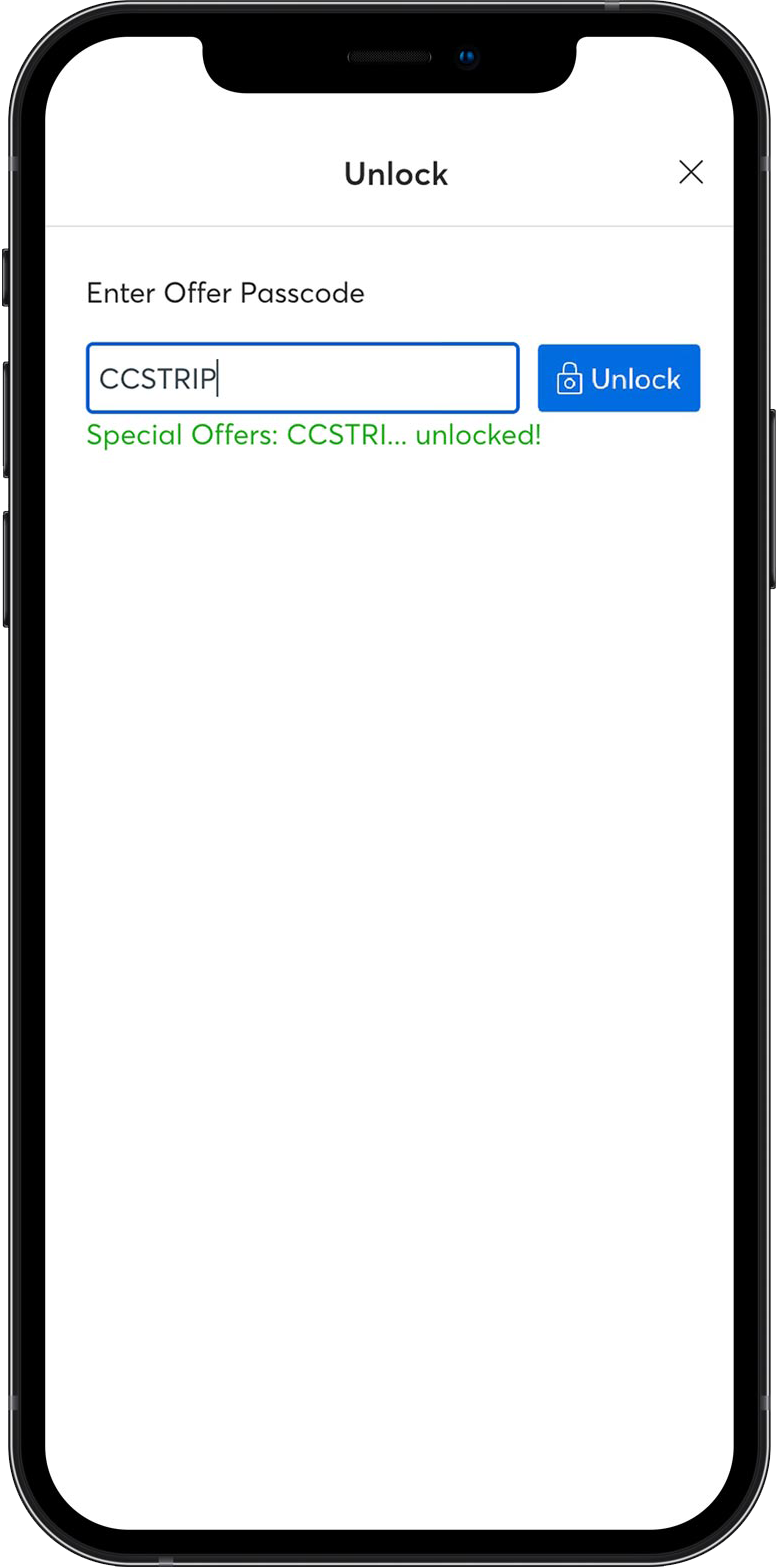The image displays a smartphone screen with a predominantly white background. The focal point of the image is the phone's camera, highlighted by a small blue dot positioned in the center of the screen. Above this, there is an oval shape where the speaker is located. The top of the screen features the word "UNLOCK" in bold, black, uppercase letters. To the right of this text is a black "X". Below these elements runs a thin gray line that stretches horizontally across the screen.

Beneath the gray line, the words "ENTER OFFER PASSWORD" are written consecutively in black, uppercase letters, each word starting with a capital letter. There is a blue-outlined box containing the text "CCSTRIP" in black, uppercase letters. Adjacent to this box is another blue box with white font that reads "UNLOCK", accompanied by a white lock icon.

Further down the screen, in green text with capitalized first letters, appears "SPECIAL OFFERS...", with "CCSTRI..." following, all written in uppercase letters. Near the bottom of the screen, the word "UNLOCK!" is prominently displayed with an exclamation point.